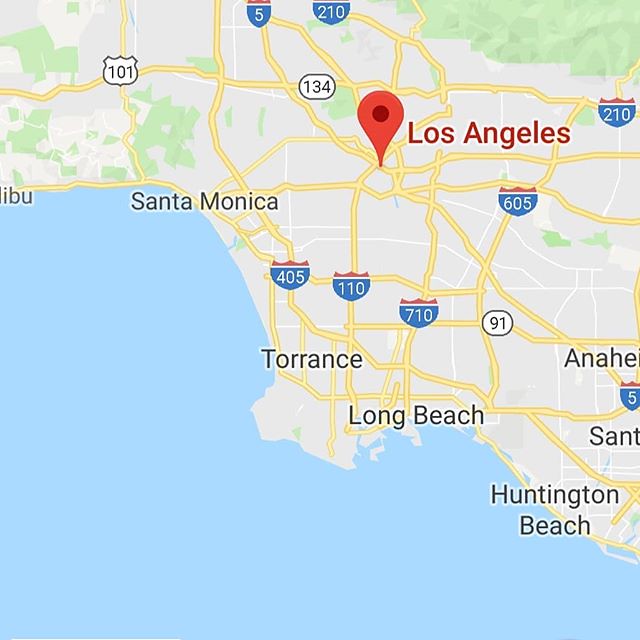This detailed map screenshot resembles the interface of an iPhone Maps application, displaying a focused view of California with emphasis on Los Angeles. A prominent red pin marks Los Angeles, surrounded by a network of yellow lines representing major highways, including the 405, 110, 710, 605, and 210. Additionally, white symbols denote other highways such as the 101 and 134. Various locations are labeled, including Santa Monica, Torrance, Long Beach, Huntington Beach, and partially visible names like Anaheim and Santa Ana (indicated by the starting letters "S-A-N-T"). The upper right corner features a green area, likely representing a park or natural reserve, while the bottom left and right edges of the map are bordered by the coastline, highlighting the proximity to the Pacific Ocean.